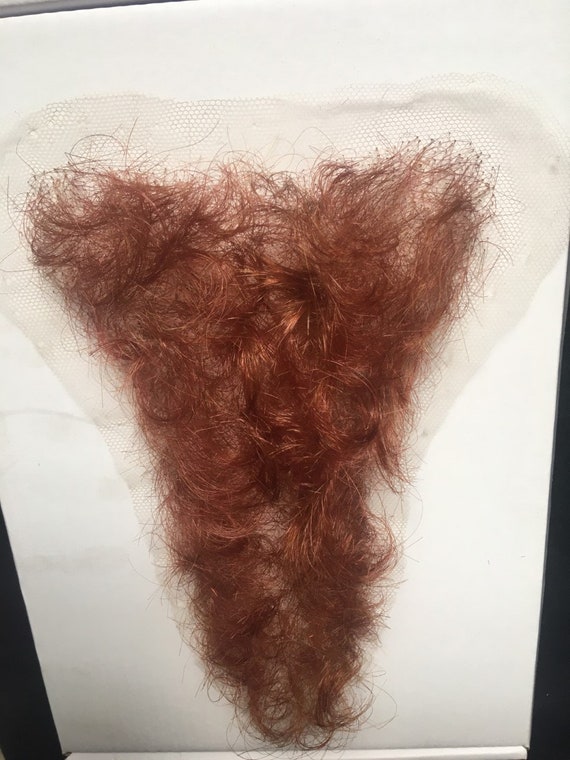The image features a white background with small patches of black in the left corner and right-hand side. Against this backdrop is a triangular-shaped bandage-like object, which appears to be made of a porous material that allows air and water to pass through. Attached to this bandage is a thick cluster of brownish-red, curly hair that has a slightly frizzy texture. The hairs seem to have been randomly cut or pulled off, suggesting they might have been removed from a hairy part of the body. The overall shape resembles a wig, set in a way that could imply it being used for a body part rather than the head, possibly indicating an unconventional use or an artistic setup. The hair strands are visibly attached to a lace front, enhancing the detailed texture of the curls in the image.